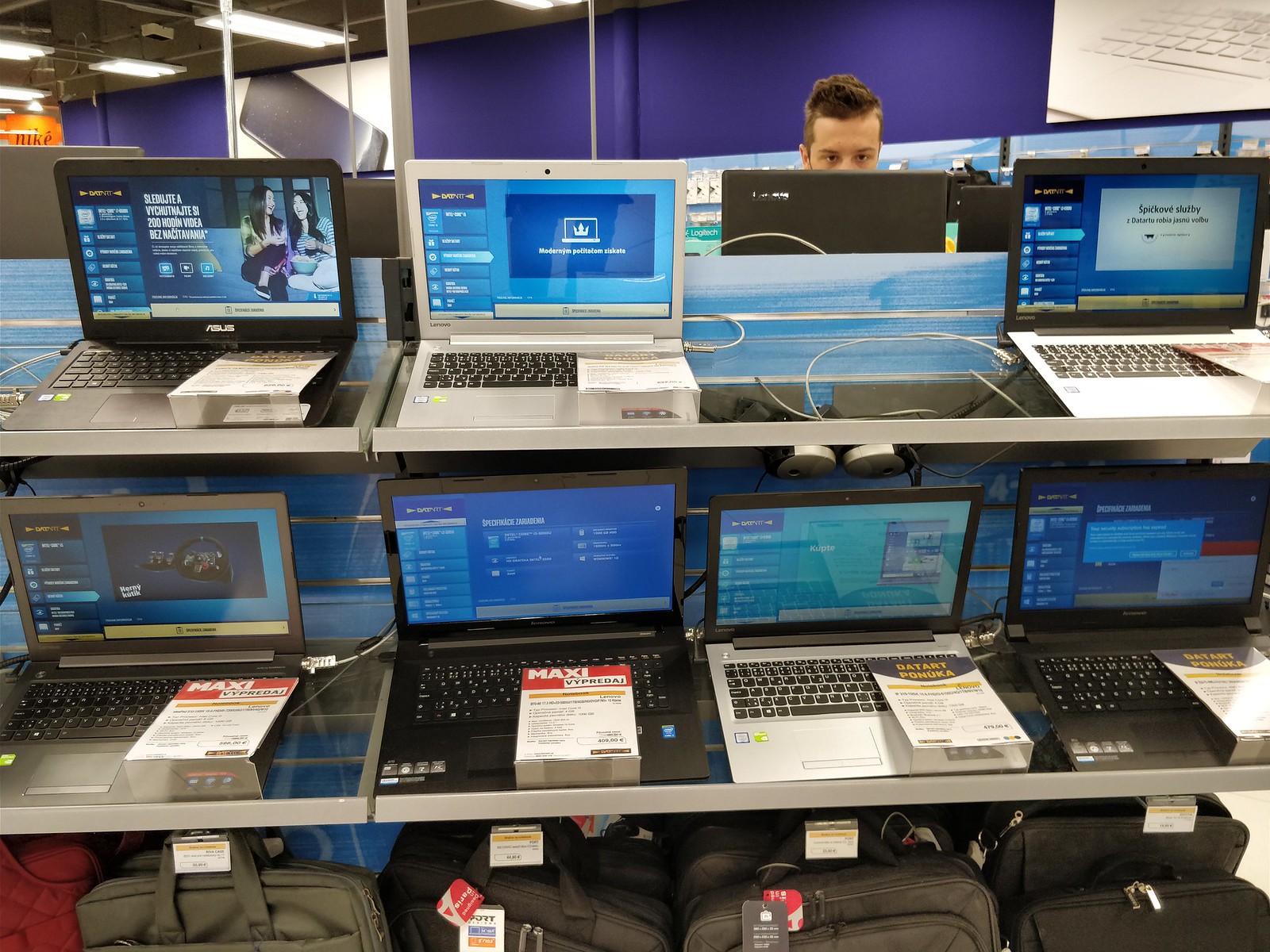An early 20s male, possibly 19, is standing in an electronics store, deeply engrossed with a laptop whose cover is flipped up, suggesting he's concentrating on a task. He's surrounded by an array of at least eight different laptops displayed on shelves, each accompanied by informational cards detailing their specifications. The shelves are organized with two rows of laptops, the top rows showcasing various brands with characteristic Intel and NVIDIA stickers, albeit in different languages, suggesting an international setting. The laptops are secured with chains or locks. Below these shelves, there's a variety of laptop bags in different shapes, colors, and sizes, including red, grey, light grey, and black. The store features an orange and purple background with large fluorescent lights, creating a brightly lit environment. A male with brownish hair can be partially seen peering over the opposite side of the shelving, with only his eyes, hair, most of his nose, and ears visible, indicating his interest in the laptops as well. The electronics store also prominently displays a Nike sign in the background.